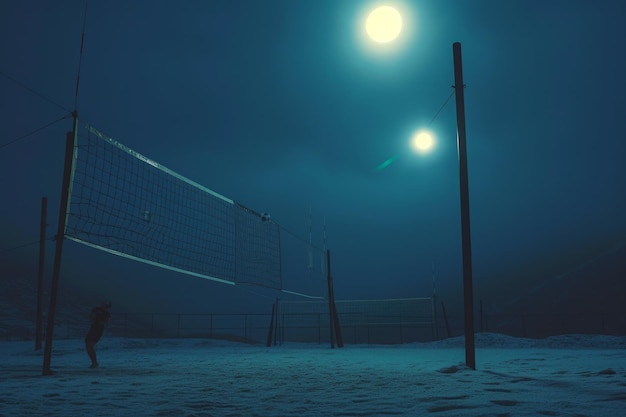The image is a landscape-oriented photograph of a nighttime outdoor volleyball setting with a prominent blue hue. The foreground features a sand volleyball court, marked by two vertical metal poles that nearly reach the top of the image and support a volleyball net extending from the left side to the center. To the right side of the image, there is an additional pole and a soccer net visible towards the edge. The scene is illuminated by a streetlight on the right, casting light on the net and the surroundings, contributing to the bluish tint that pervades the photograph.

A black silhouette of a person is visible under the net, appearing to be in the act of hitting a volleyball over it. The nighttime ambiance is further emphasized by the presence of a moon high in the sky and a smaller, second moon-like light below it, adding to the surreal quality of the scene. In the background, faint hills or mountains are partially obscured by fog, enhancing the mysterious, deep gray contrast of the image.